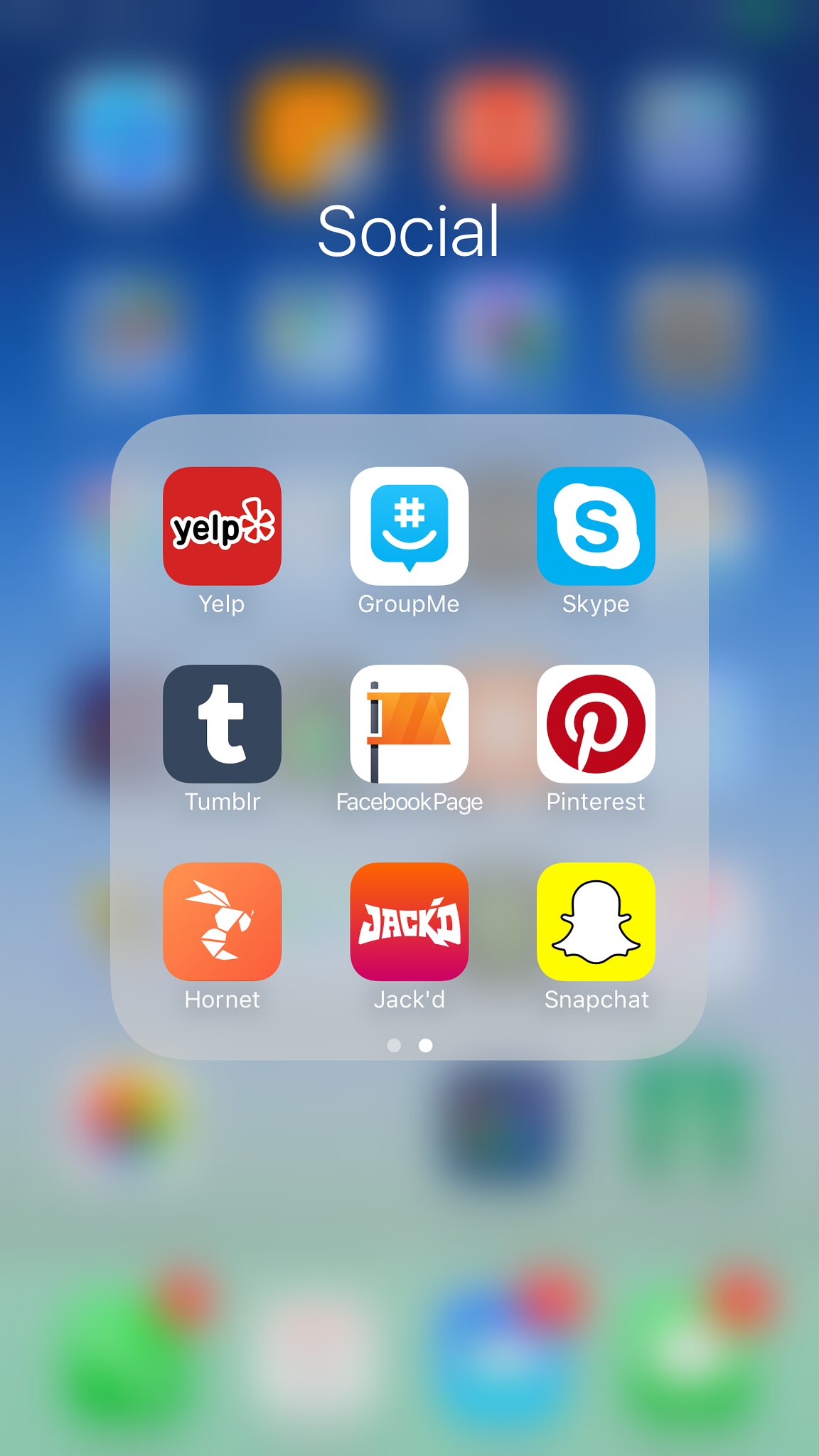A smartphone screen with a blurry background displays a neat 3x3 grid of vividly clear and sharp app icons in the foreground. Starting from the top left, the first row features the red Yelp icon, followed by the blue GroupMe icon, and the blue Skype icon. The second row begins with an unidentified app represented by a "T" (referred to as "Tee"), followed by the Tumblr icon with its distinctive white "T" on a black background, and the Facebook Pages app icon depicted as an orange flag. The third row includes the Hornet app, followed by Jacked, and finally the yellow Snapchat ghost icon. Despite the out-of-focus screen showing multiple apps, these nine icons stand out prominently, offering a clear snapshot of this segment of the user's home screen.